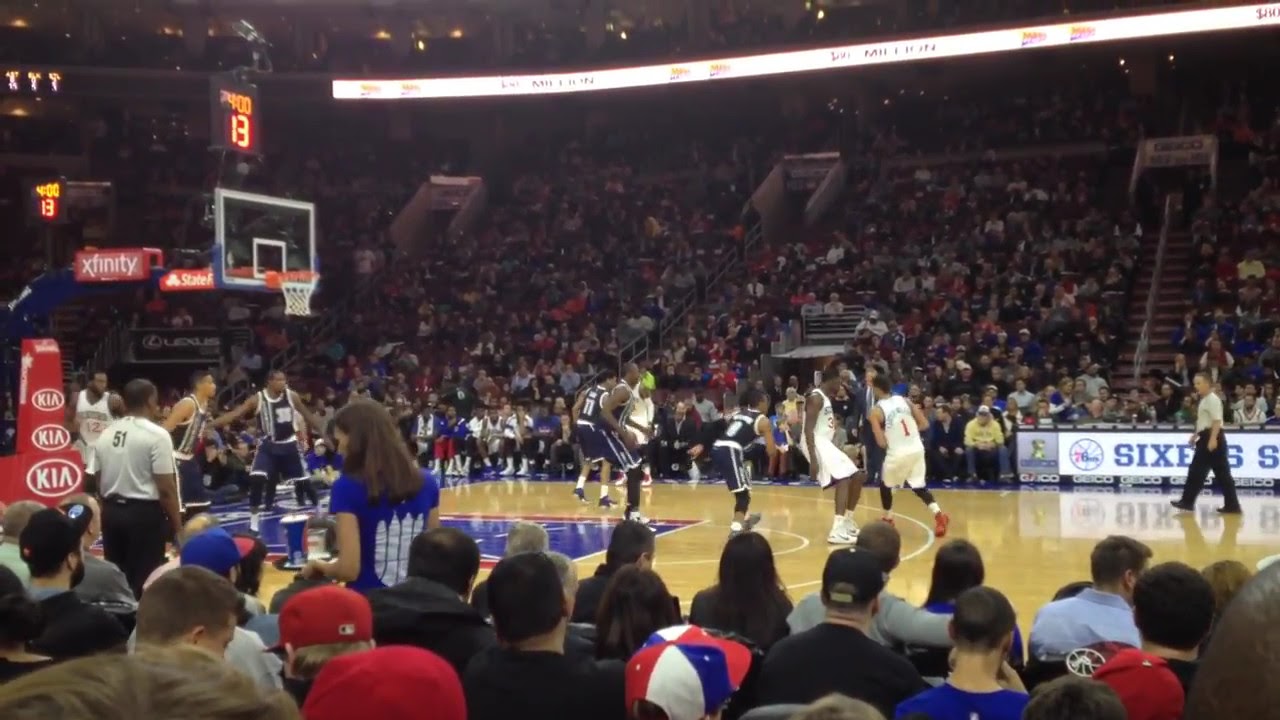The photograph captures an intense, professional NBA basketball game from a viewpoint close to court side, providing a clear, detailed representation of the on-court action and ambiance. The horizontally-aligned rectangular image features players from two teams: one team in navy blue uniforms with white numbers, the other in white uniforms. The court itself boasts a light, highly polished wooden floor with a blue painted area under the hoop, which is situated in the upper left corner with the number "13" in orange and "4:00" displayed above it.

The stands are packed with spectators, many of whom are wearing red ball caps. The audience appears captivated, focusing intently on the game. Visible sponsors include prominent red logos for Kia and Xfinity alongside other advertisements, though some, like State Farm and another partially-visible "Lex," are less discernible.

Additionally, on the opposite side of the court, there's a large "Sixers" banner, indicating that the Philadelphia 76ers are one of the teams playing. Other notable elements include two visible referees on the court officiating the game and the overhead lighting which brightly illuminates the entire scene. The vibrant atmosphere and close-up perspective encapsulate the thrilling essence of live professional basketball.